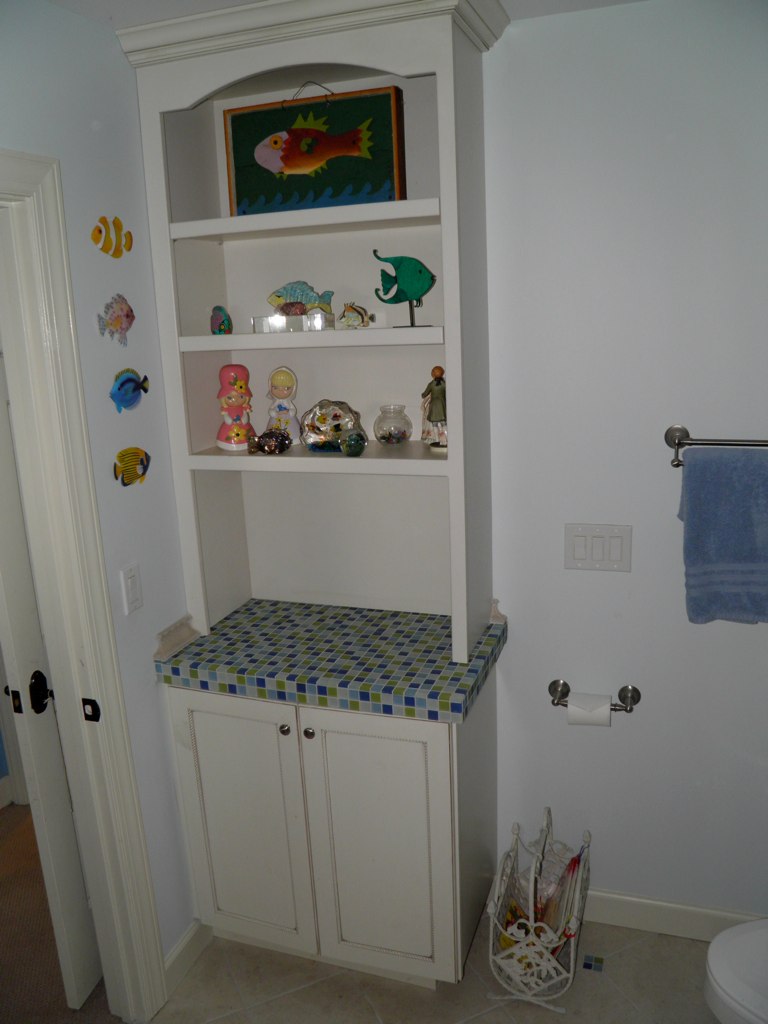The image features a corner bathroom setup designed for children, characterized by a white cabinet paired with shelving. The cabinet includes a countertop made from blue and gray mosaic tiles, adding a touch of vibrant detail to the room. The shelves, painted in white, extend from the top of the cabinet all the way to the ceiling, curving into an arch at the top.

Positioned against the right wall, the cabinet is nestled neatly into the corner. On the wall adjacent to the shelving are four fish figurines, arranged vertically one above the other, adding a playful, aquatic theme to the space.

To the left of the cabinet, a toilet paper holder is mounted on the wall, holding a partially used roll. Below this, a wicker magazine rack sits on the floor, offering a rustic touch. Slightly above and to the right, a towel holder is attached to the wall, adorned with a neatly folded blue towel.

In the bottom right corner of the image, the edge of a toilet is visible, suggesting the practical and compact layout of this child-friendly bathroom.